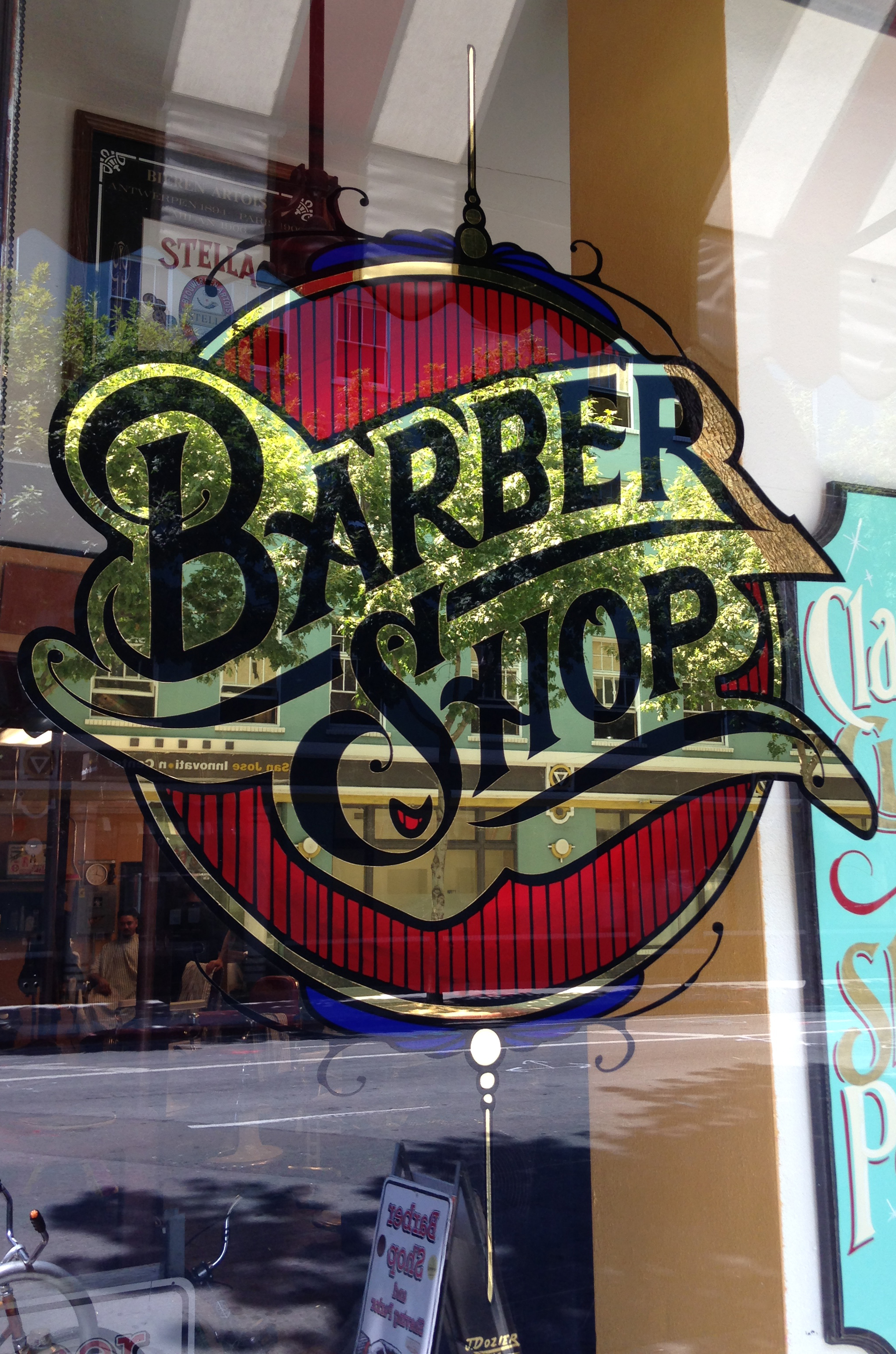This is an image of a barbershop's front window featuring an ornate, circular red logo with black and gold typography that reads "Barbershop." The black text uses negative space to create a translucent effect, allowing glimpses of the interior through the window. The logo is complemented by scrawly cursive writing with "Barber" at the top and "Shop" beneath, each word underscored by black lines. Additional colors in the scene include white and baby blue elements that enrich the design. To the right of this primary logo is a small, partially visible sign in coordinating shades of red, blue, and gold. Inside the barbershop, which appears quite upscale, are attractive stools and various other signs, including one prominent sign reading "Stella." The overall aesthetic suggests a place of refinement and style.